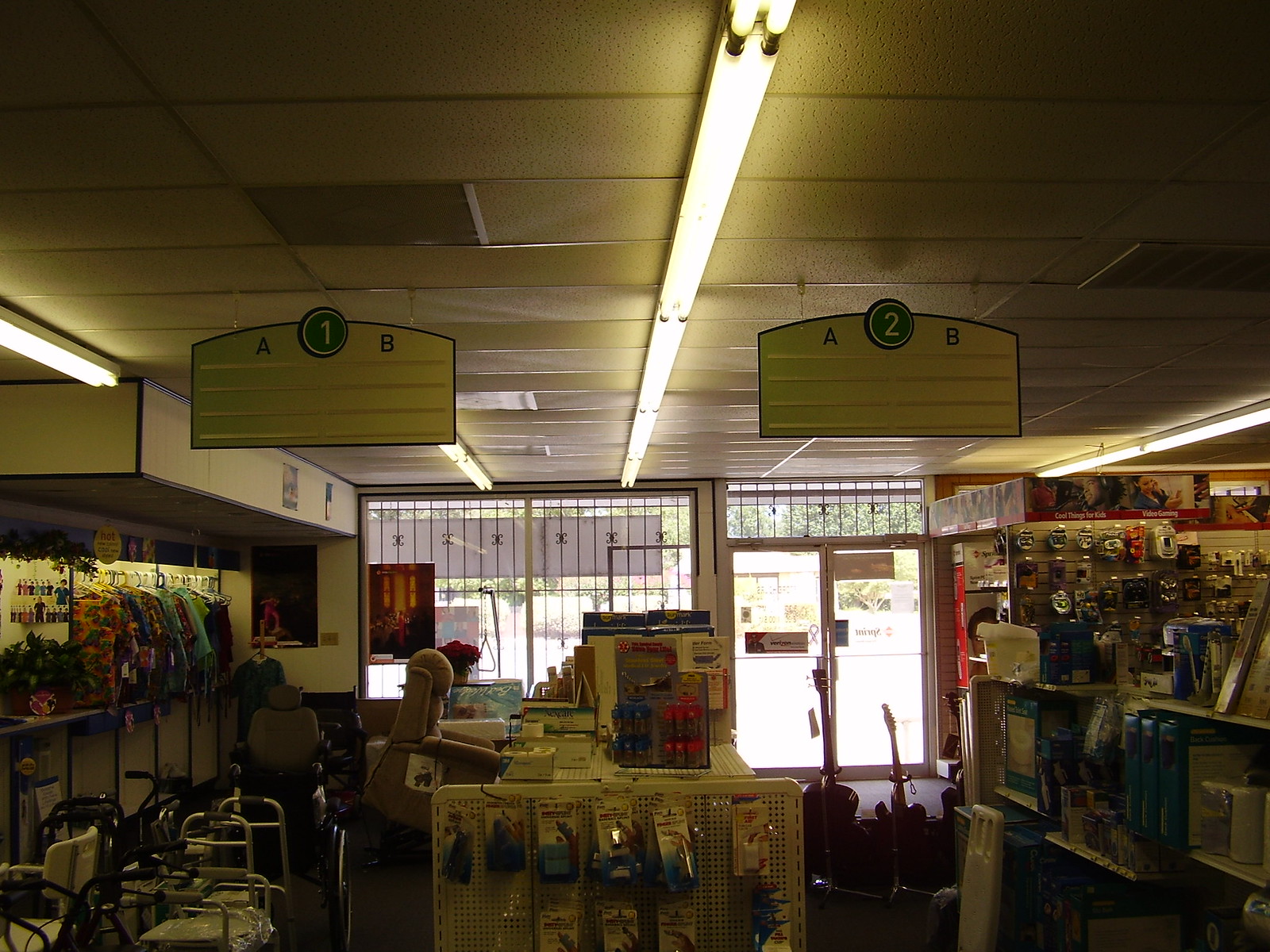In this blurry color photograph depicting the interior of a store, the focal point is the spacious front window and door, which feature large glass panes bordered with white framing. The door is actually a double door with glass panes and a transom window above it. Suspended from the ceiling are two rectangular signs with an arc-like top, labeled "1AB" and "2AB," but lacking further information on aisle content.

The store is well-lit by white fluorescent lights on the ceiling, adding to the clarity of various sections despite the overall blurriness. To the left, there's a shelf holding baby clothes, and beneath it, an assortment of medical mobility aids, including walkers, shower chairs, and canes. Additionally, a recliner and clothing rack are visible in this area.

Towards the center-left foreground, there are recliners and an array of objects hanging on a pegboard, although their specifics are unclear. On the right side, beneath the window, there's a shelf displaying electronics and an office chair situated behind a checkout counter. Metal grills secure the windows, ensuring safety. This comprehensive setup showcases a diverse range of products from clothing to electronics, emphasizing the store's wide variety of merchandise.